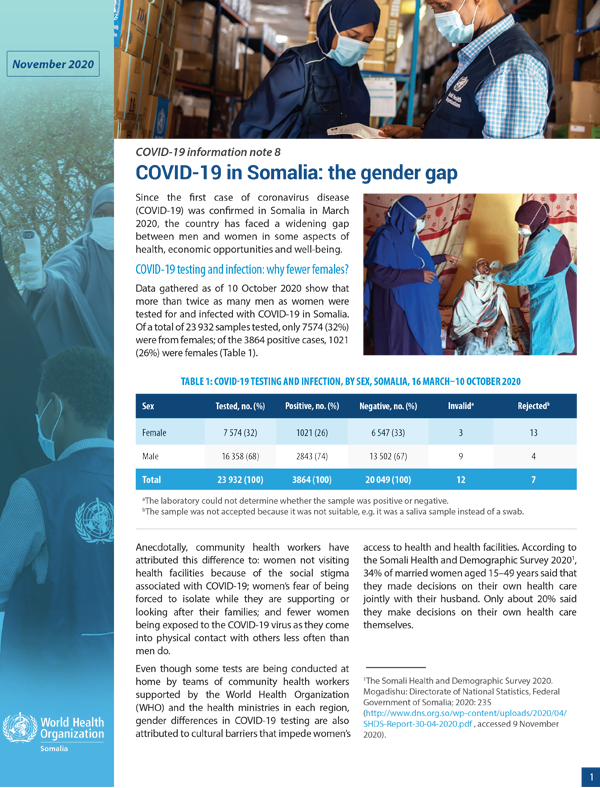This is a screenshot from the World Health Organization Somalia, dated November 2020. A vertical banner with a blue hue runs down the left side of the page. On the banner, a woman wearing a hijab and a face mask is depicted holding a touchless thermometer. She is pointing the thermometer towards the left. Below her, a man wearing a mask, a blue shirt, and a blue vest with the World Health Organization logo on the back, is facing away from the camera.

At the bottom of this vertical banner, the World Health Organization logo is displayed along with the text "World Health Organization Somalia." 

The top of the page features a horizontal banner. This banner shows a woman dressed in dark blue attire with a matching head covering and face mask. She is facing slightly towards the right and looking downwards. To her right, a man wearing a face mask, with light skin and a blue and white checked shirt under a blue vest, faces towards the left.

Below the horizontal photo, there's a headline that reads: "COVID-19 Information Note 8, COVID-19 in Somalia, the gender gap."